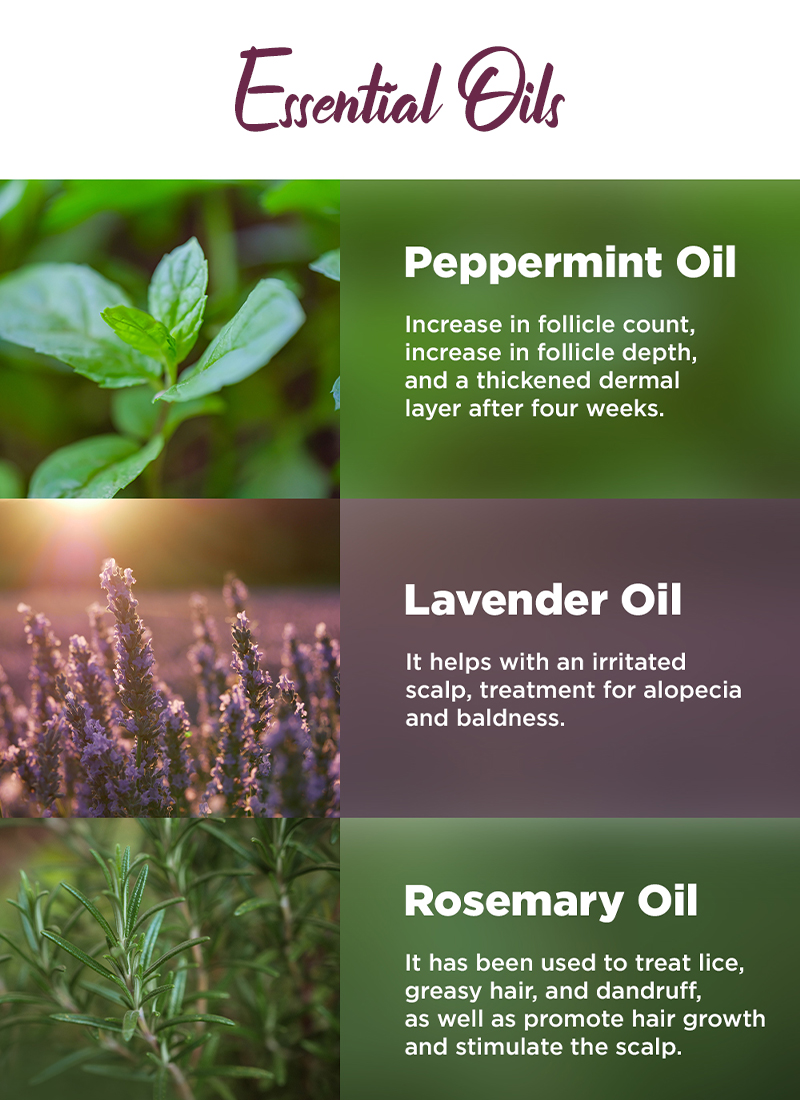The advertisement for essential oils features a prominent heading in a purplish cursive font that reads "Essential Oils," set against a white background. Below the title, the layout is divided into three sections, each dedicated to a different type of essential oil—peppermint, lavender, and rosemary—all arranged in a series of six boxes.

On the left side of the layout, there are images of the respective plants, each in its own designated box:
1. At the top left, there is an image of a peppermint plant.
2. Directly below the peppermint, the middle left box features lavender.
3. The bottom left box displays rosemary.

Adjacent to each plant image, on the right side, are corresponding boxes with details about the oil extracted from each plant:
1. The top right box, with a green background and white font, provides details on Peppermint Oil. It reads: “Peppermint Oil increases follicle count, increases follicle depth, and thickens the dermal layer after four weeks.”
2. The center right box, with a lavender background and white font, describes Lavender Oil, stating: “Lavender Oil helps soothe an irritated scalp and is a treatment for alopecia and baldness.”
3. The lower right box, with a green background and white font, outlines the benefits of Rosemary Oil. It reads: “Rosemary Oil has been used to treat lice, greasy hair, and dandruff, as well as to promote hair growth and stimulate the scalp.”

Together, these sections provide a detailed and organized overview of the benefits and uses of these essential oils for hair care.